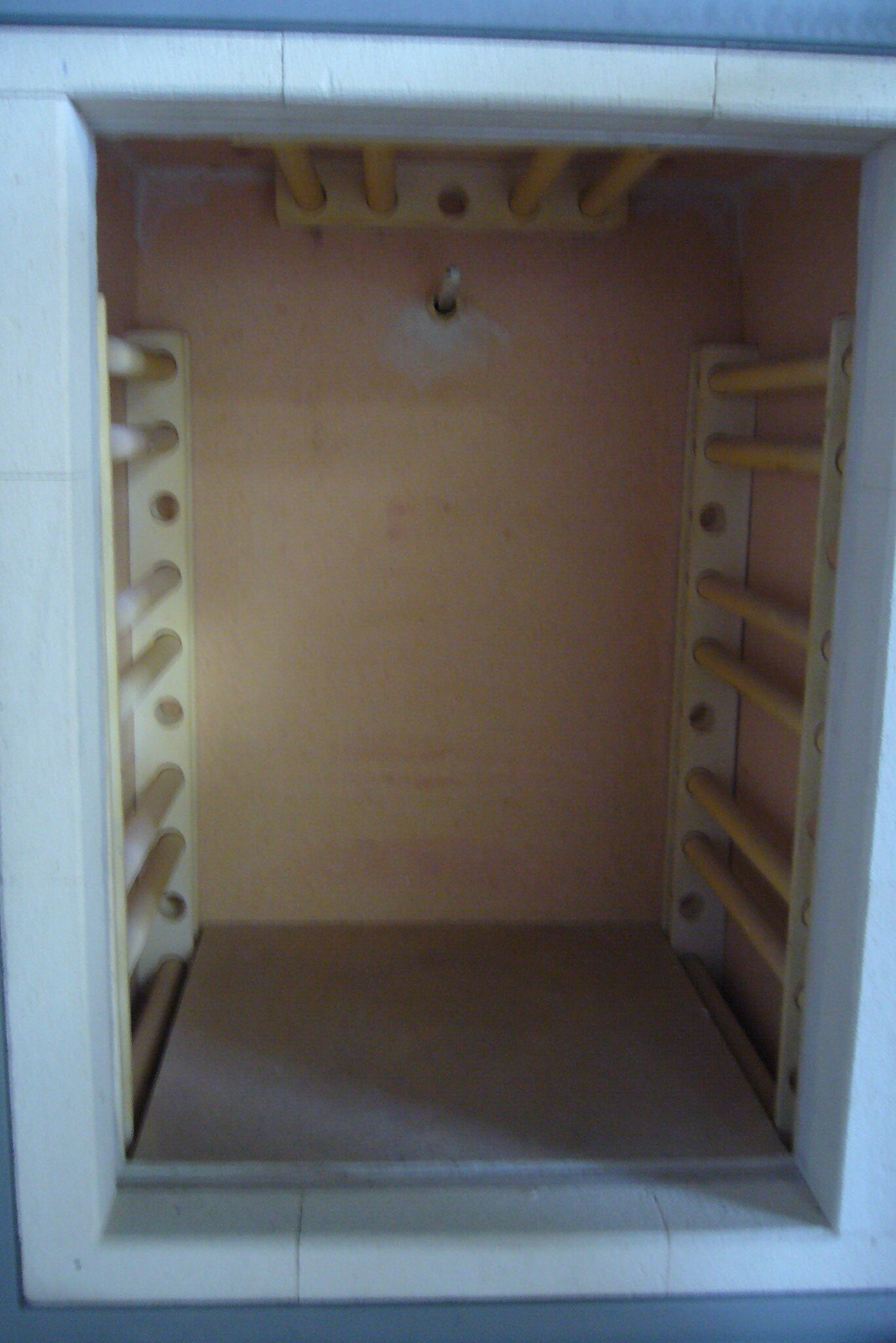The image captures a storage space nestled within a recess framed by gray bricks and featuring an open entryway with no door. The walls and floor are constructed from light-colored plywood, tightly sealed at the corners and edges with white caulking. The unit is enveloped in a light blue border on the outside, transitioning to darker blue toward the top. Inside, the space is relatively shallow, approximately five feet deep and eight feet tall, forming a vertical rectangular shape. The base has a grayish hue.

Inside the unit, mounted on the ceiling, left wall, and right wall, are multiple cylindrical wooden rods, arranged in two racks at consistent intervals. The left and right walls each feature two white rectangular bars vertically positioned in the corners, facilitating the placement of these rods. The rods are organized in pairs, interspersed with empty spaces, creating a pattern: one rod, skip one space, two rods, skip one space, and so on, culminating in nine to ten positions. This arrangement reaches about three-fourths of the way up the walls. On the ceiling, the rods follow a similar pattern but run horizontally across the unit. The ceiling rack includes five positions, with four occupied by wooden rods and a gap in the middle. The back wall is light brownish and plain, maintaining the minimalist design of the storage space.